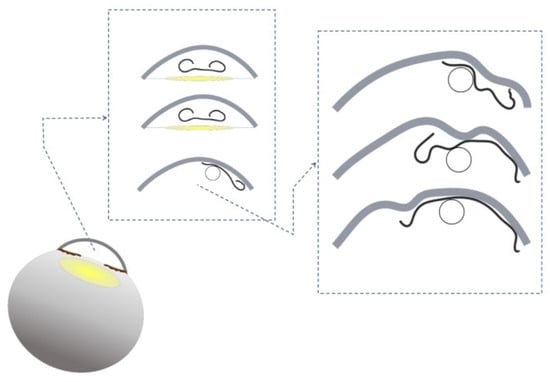The illustrated diagram begins with a gray oval in the bottom left corner, which appears to represent an eye, featuring a flat top edge. Beneath this flat edge is a small yellow oval, topped by a black outline of a half dome from which two brown lines extend parallel to the flat edge. A dotted black line emerges from this setup, arcing up to the left before pointing right towards a vertically outlined rectangle. This rectangle contains several intricate designs: three gray half domes at the top, each with yellow ovals and black lines inside. The black lines resemble a curled horseshoe on one side, leading to a more tightly curled section on the right. The third dome is similar but includes a circle on the right with a crowbar-like line above it. The diagram continues with another arrow pointing to a second outlined rectangle on the right, which showcases an expanded view of the third dome. Here, the dome is indented on the top right, and the yellow oval is removed, possibly illustrating a transformation or detail about the structure. The background of the image is white, and the color scheme primarily uses gray, black, and yellowish-green hues. The overall visual seems to depict a zoomed-in examination of eye components or a follicle-like structure, with progressive magnification and detailing through each section of the diagram.